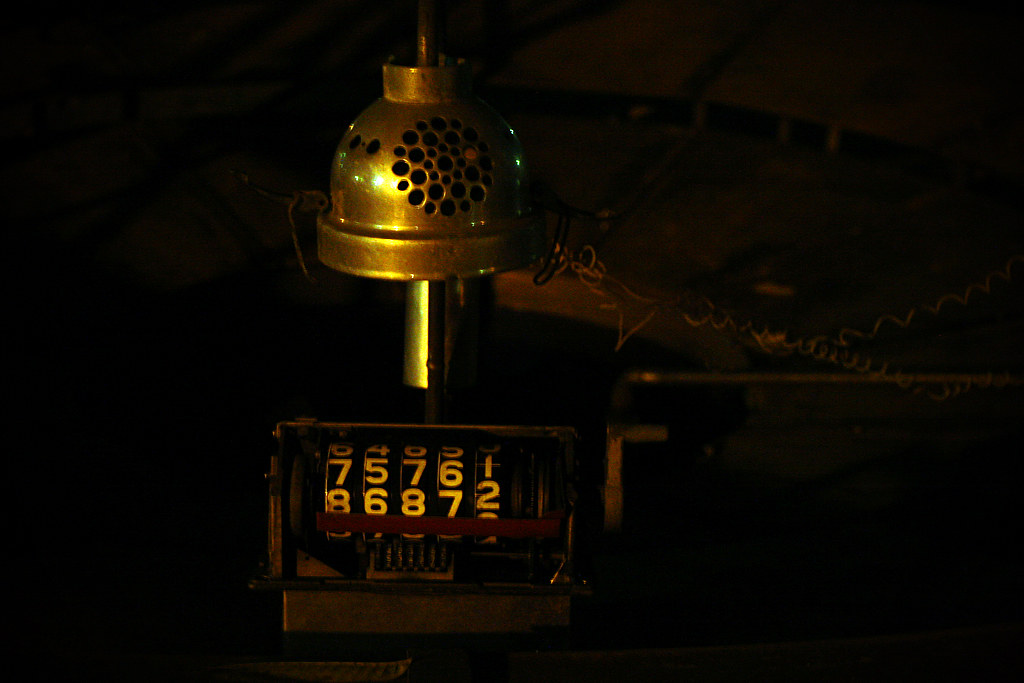An old, antique mechanical counter is poorly illuminated in this very dark photograph. The counter, possibly situated on a surface, features a prominent bell covering on top. The device appears quite aged, almost rustic. Visible are two distinct lines of numbers on rotating dials: the first line reads 7576 transitioning to 2, while the second line reads 8687 transitioning to 3. The overall details are obscured by the darkness, making it difficult to discern additional elements, though there is a faint indication of a possible cord or elastic nearby.